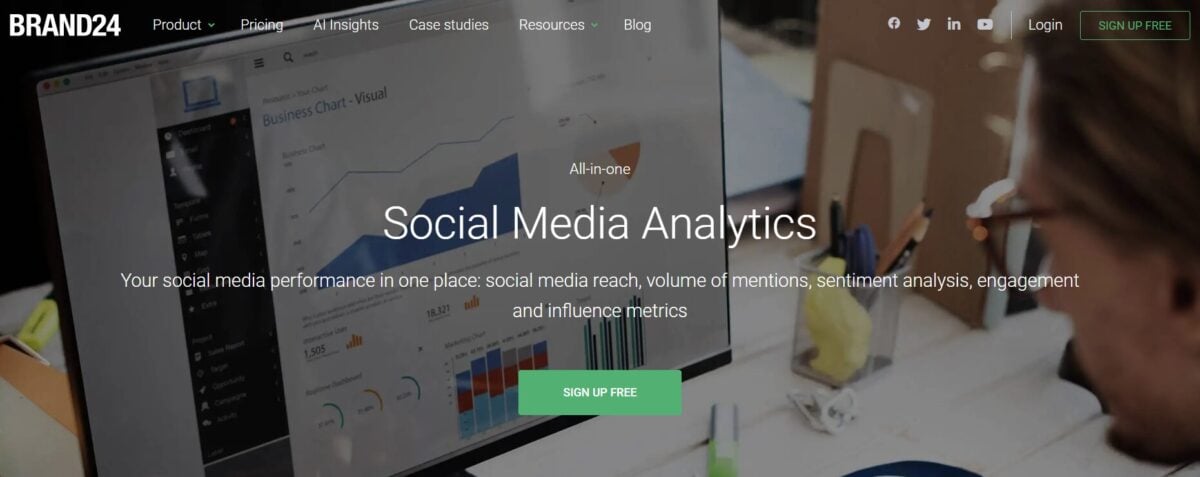The image is a landscape-oriented screenshot depicting a person working in an office setting. On the right side of the image is a light-skinned individual with blondish, dirty brown hair, wearing glasses and sporting a goatee. The person is intently looking at a computer screen, engrossed in their work. In the office, a pencil holder, paper clips, and a collection of folders and documents organized in a book holder are visible.

The computer screen showcases a detailed interface of a business analytics platform called "Brand 24." The upper left corner of the screen features the "Brand 24" logo, while the top navigation bar includes tabs labeled "Product," "Pricing," "AI Insights," "Case Studies," and "Resources," along with a "Blog" link. In the upper right corner, icons for social media platforms such as Facebook, Twitter, LinkedIn, and YouTube are displayed beside a "Login" button and a prominent green "Sign Up Free" button.

The main content of the screen highlights various sections of social media analytics. A tiny font in the middle of the screen reads "All-in-one," while larger text below prominently states "Social Media Analytics." The accompanying slogan beneath, "Your social media performance in one place," is followed by a list of analytic features including "Social media reach," "Volume of mention," "Sentiment analysis," "Engagements," and "Influence metrics." At the bottom of this section, another green "Sign Up Free" button is displayed in small font.